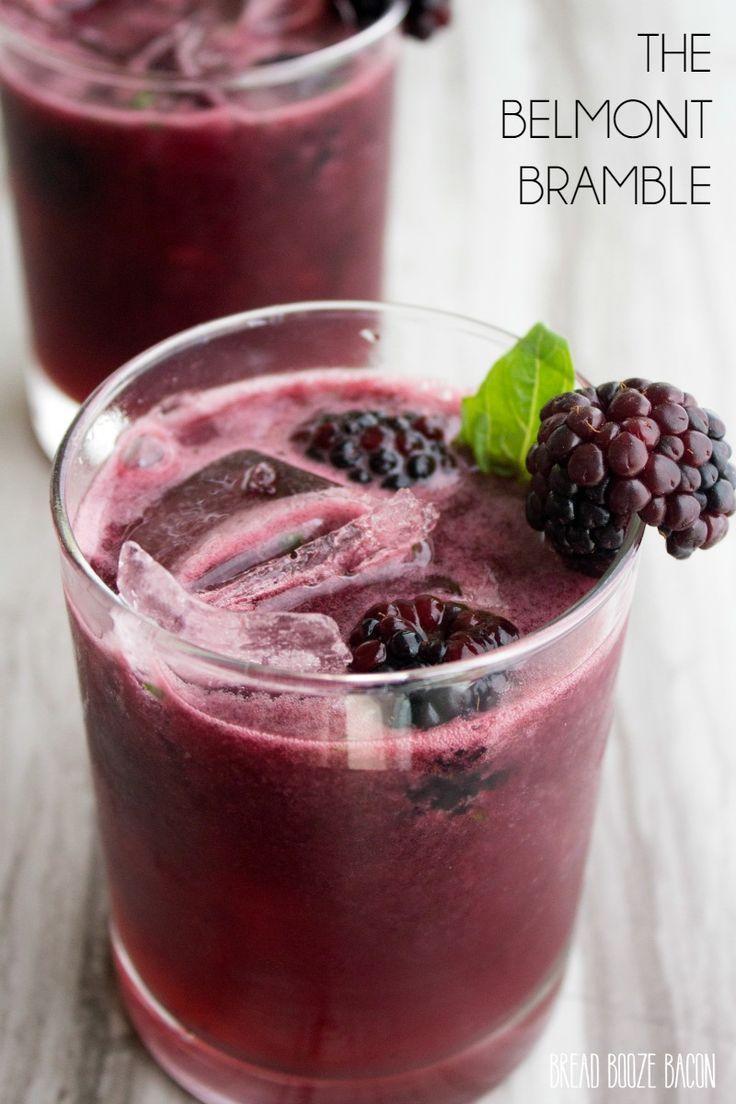In this photorealistic image, the focal point is a clear tumbler glass filled with a dark purple, non-transparent liquid that appears slightly carbonated. The glass, taking up most of the foreground, is garnished with ice cubes, floating blackberries, and a sprig of mint. Another blackberry decorates the rim of the glass. Behind the main drink, slightly out-of-focus, is a second similar glass, hinting at a second serving. The background features a light laminate wood color, emphasizing the vibrant hues of the beverages. In the top right corner, black text reads "The Belmont Bramble," suggesting the name of the drink or the establishment. In the bottom right corner, white text against the light background states, "Bread, Booze, Bacon," indicating a possible association with the venue or the type of offerings available. This image, likely an advertisement, showcases a delicious, visually appealing drink, perfect for a refined yet casual setting.